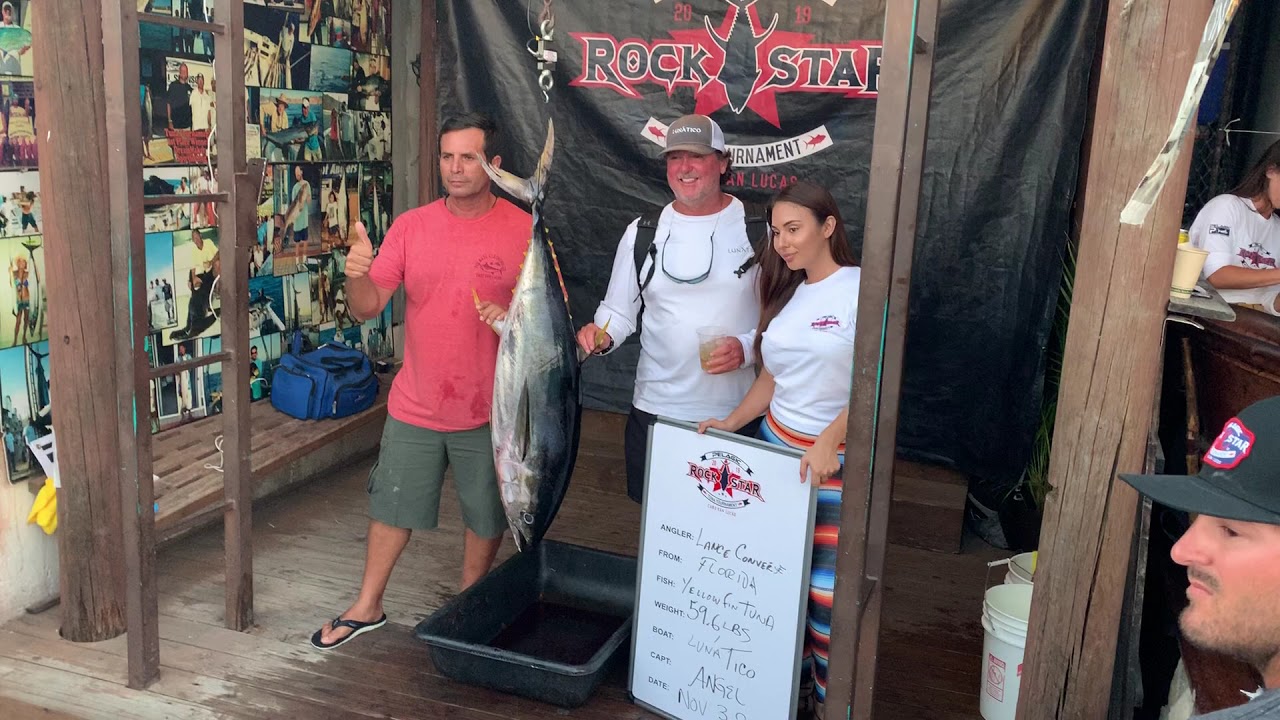In this vibrant and detailed color photograph, five people are gathered at a fishing competition booth, posing proudly. Central to the image are three individuals standing beneath an elaborate pulley system hoisting an impressive fish. On the far left stands a man with dark hair, dressed in a coral-colored t-shirt, green shorts, and black flip-flops, his hand gripping the fish while he gives a thumbs-up. The man in the middle, wearing a long-sleeve white shirt, a gray and white cap, and sunglasses around his neck, smiles broadly, also holding the fish. To the right is a young woman with long dark hair, clad in a white t-shirt with a small red "Rockstar" logo and vibrant, multicolored striped pants. She holds a white board detailing specifics about the catch, including the angler, Lance Convert from Florida, a yellowfin tuna weighing 59.6 lbs, caught from a boat named Luna Tico, Cape Angel, dated November 30th. Behind them, a black curtain prominently displays the "Rockstar Tournament" logo with a stylized upside-down fish. The setting appears to be a wooden pier, adorned with various bait and tackle supplies. Off to the top right, a person with long hair and a white shirt with red text is seated behind a counter, while another individual in the bottom right corner, wearing a black baseball cap with a red and blue logo and a gray t-shirt, observes the scene.